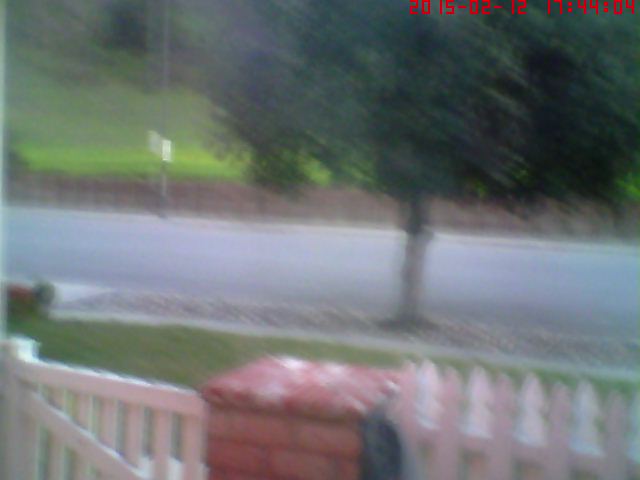A blurry, grainy color photo dated 2015-02-12-17-44-04 shows an overcast day with a view from a porch. Dominating the middle of the image, a large tree with a light brown trunk stands tall, surrounded by a patch of grass in a gravel area. In the foreground, a white picket fence with a small gate and a short brick pillar is visible. Beyond this, the yard appears small, leading to a narrow street. Across the road, a strip of sidewalk and more green grass transitions into rolling green hills, adding a quaint, picturesque charm to the scene.